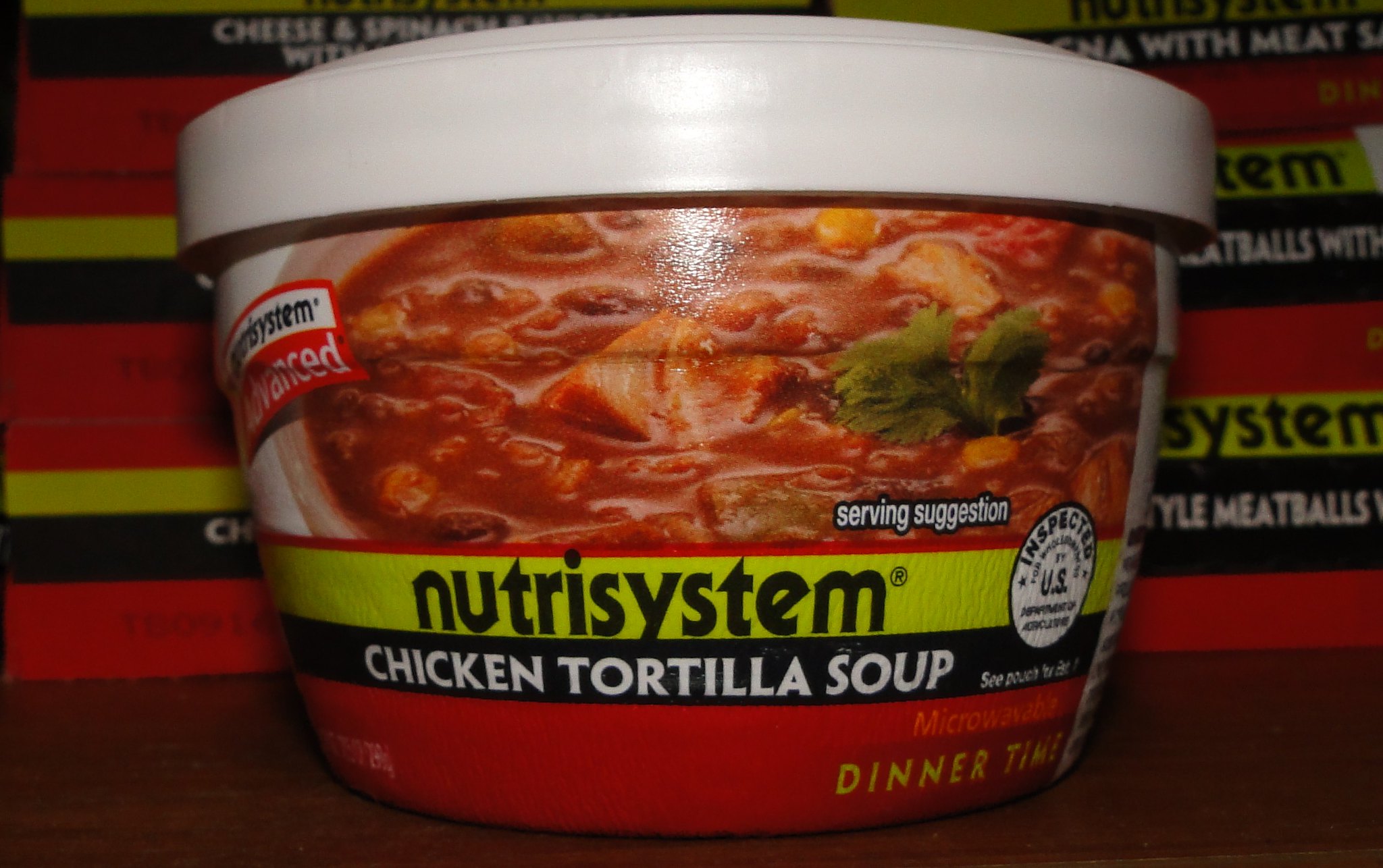**Detailed Caption:**

The image features a single-serve Nutrisystem instant soup bowl, specifically the Chicken Tortilla Soup variety. The bowl has a prominent white plastic lid and a compact shape typical of soup containers. A vacuum-sealed wrapper encloses the bowl, showcasing an appetizing photograph of the soup. The Nutrisystem branding is evident, with "Nutrisystem Advanced" noted in the upper left corner. A large green horizontal stripe across the container bears the Nutrisystem name in black lettering, while a black stripe beneath it indicates "Chicken Tortilla Soup" in white letters.

Additional details include a quality assurance mark in the lower right-hand corner, indicating that the soup is inspected and authorized, possibly by a U.S. regulatory body. The packaging also highlights that the soup is microwaveable and suitable as a dinner option, as denoted by the "Dinner Time" text.

In the background, several boxes of Nutrisystem meals are visible. Among them, three boxes are discernible, one of which mentions meatballs, alongside another depicting cheese and spinach, adding context to the Nutrisystem meal lineup.